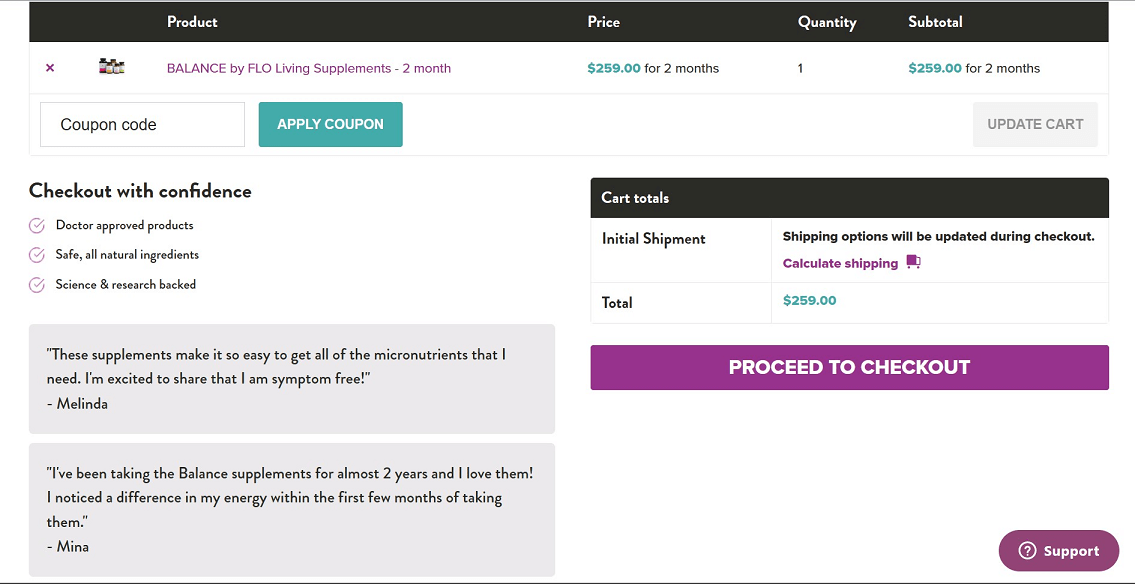This image is a screenshot from a webpage displaying a product purchase summary. At the top of the page, there is a black, rectangular banner with the word "Product" on the left. Moving towards the center, it lists "Price," "Quantity," and "Subtotal" in that order.

The product being purchased is "Balance by Flow Living Supplements (Two Months)," priced at $259. The quantity is one, making the subtotal $259 for the two-month supply.

Below this summary, there is a section where users can enter a coupon code in a designated rectangle and click on a teal button labeled "Apply Coupon."

Further down, the page reassures customers with a "Check Out with Confidence" section, featuring three purple checkmarks alongside the following claims:
- "Doctor Approved Products"
- "Safe, All Natural Ingredients"
- "Science and Research-Backed"

At the bottom of the page, there are customer testimonials. One quotes Melinda: "These supplements make it so easy to get all of my micronutrients that I need. I'm excited to share that I am symptom-free." Another testimonial from Mina states: "I've been taking the Balance supplements for almost two years, and I love them. I noticed a difference in my energy within the first few months of taking them."